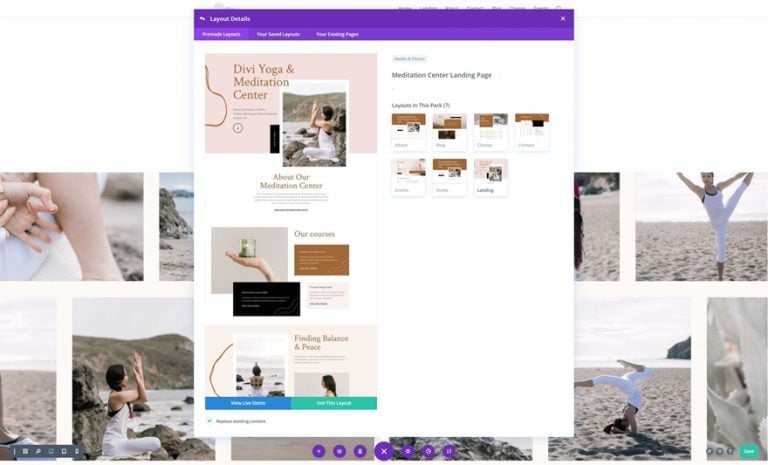The image is rectangular, orientated horizontally, with a prominent pop-up window overlaying other elements. The pop-up window features a blue header with unreadable white text and several small tabs. Below the header, a large peach-colored section displays the title "Divi Yoga and Meditation Center" along with an image of an individual meditating or practicing yoga outdoors. Additional smaller images and text are visible below this main section, including phrases like "Iowa Courses," an image of a hand holding a candle, and the words "Finding Balance and Peace." Towards the bottom of the pop-up, there are two boxes: a blue one with white text on the left and a green one with white text on the right, both situated below another "Finding Balance and Peace" text. On the right side of the pop-up, it is labeled "Meditation Center Landing Page" and contains various small images, although their details are unclear. Behind the pop-up, the background features multiple images of people meditating, practicing yoga, and scenic beach landscapes with water.